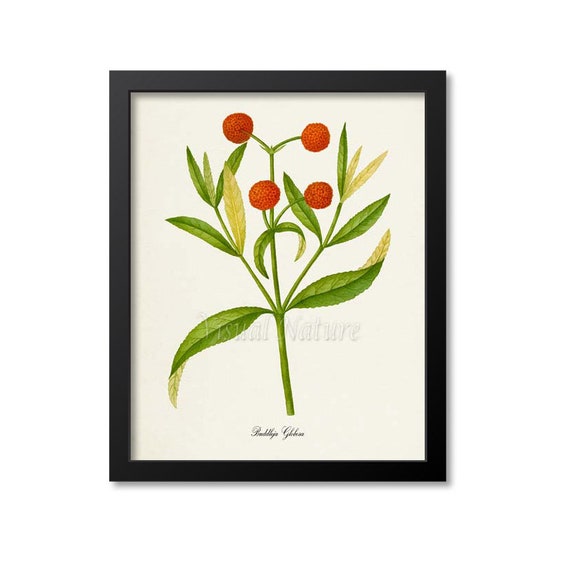Displayed in a black frame on a white wall, this small image features a detailed, symmetrical illustration or digital print of a plant. The off-white background highlights a central green stem, flanked by numerous smaller green stems and leaves. At the top center of the stem is a red berry or fruit, with a V-shaped branch extending from this point. Each end of the branch bears another red fruit, while a fourth red fruit appears slightly below and to the right of the V-branch. Two large green leaves are situated at the base of the main stem. The image includes a barely visible translucent watermark in the center that reads "visual nature." At the bottom, there is a small black label or signature, though it is too small to decipher.